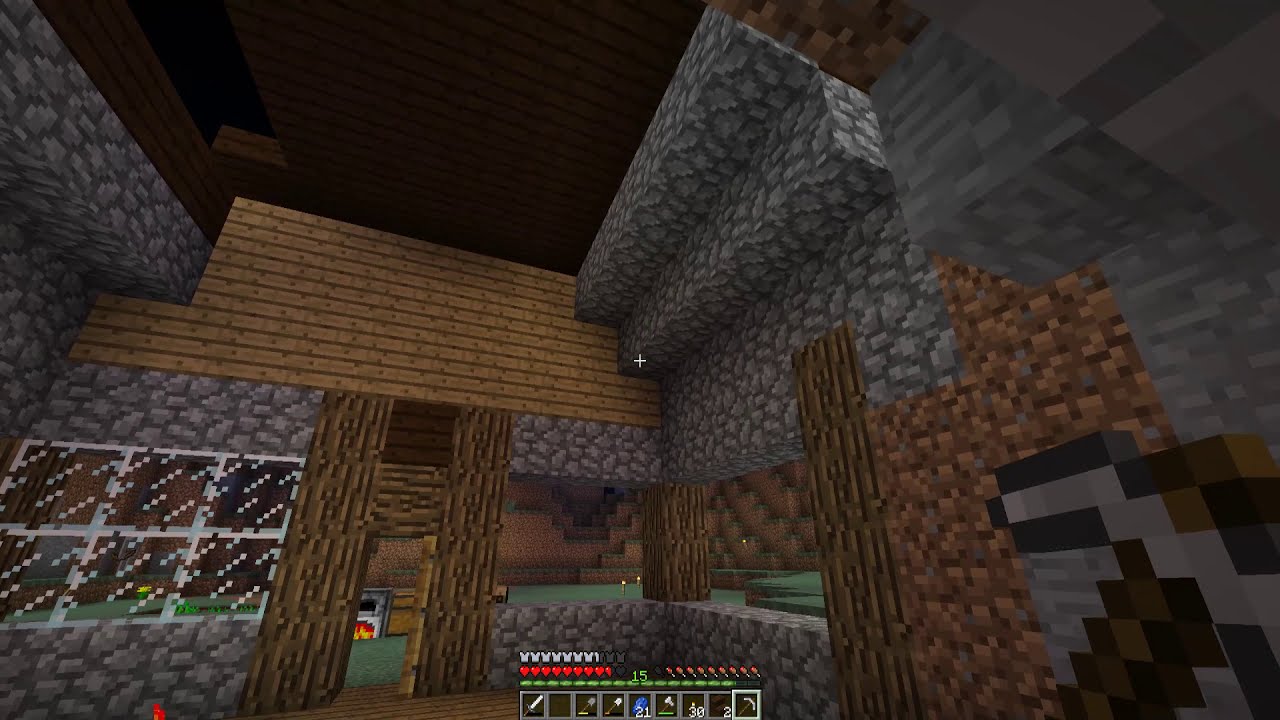The image is a screenshot taken from the video game Minecraft, showcasing an interior view of a structure that appears either player-built or pre-generated. It is a pixelated, roughly constructed building, primarily made using timber with stone foundations and some brick elements. The structure lacks symmetrical design. Visible windows and a door allow a glimpse outside, where torches are mounted on the ground and the side of a mountain, illuminating the scene.

Inside, a crafting area is seen, featuring an oven and other crafting stations. The image includes an interactive menu bar at the bottom center, displaying various tools and equipment options, consistent with typical Minecraft gameplay. The overall scene, with its mix of gray stone and brown wood textures, is rounded out by a small fire outside adding a touch of warmth and color to the otherwise muted background.